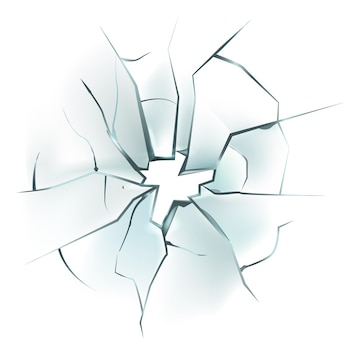The image is an illustration of shattered glass against a white background, with no border or additional elements. The glass features a distinct, jagged hole at the center, from which numerous cracks radiate outward in a pattern reminiscent of a spider's web. The artist has used shades of light gray, bluish-green, and dark green to highlight the transparency and fractured nature of the glass. The shattered effect is sharp and detailed, with horizontal and diagonal fissures branching out from the central rupture. The image, possibly a piece of stock art, has a clean white background and emphasizes the detailed, almost graphical effect of the broken glass.